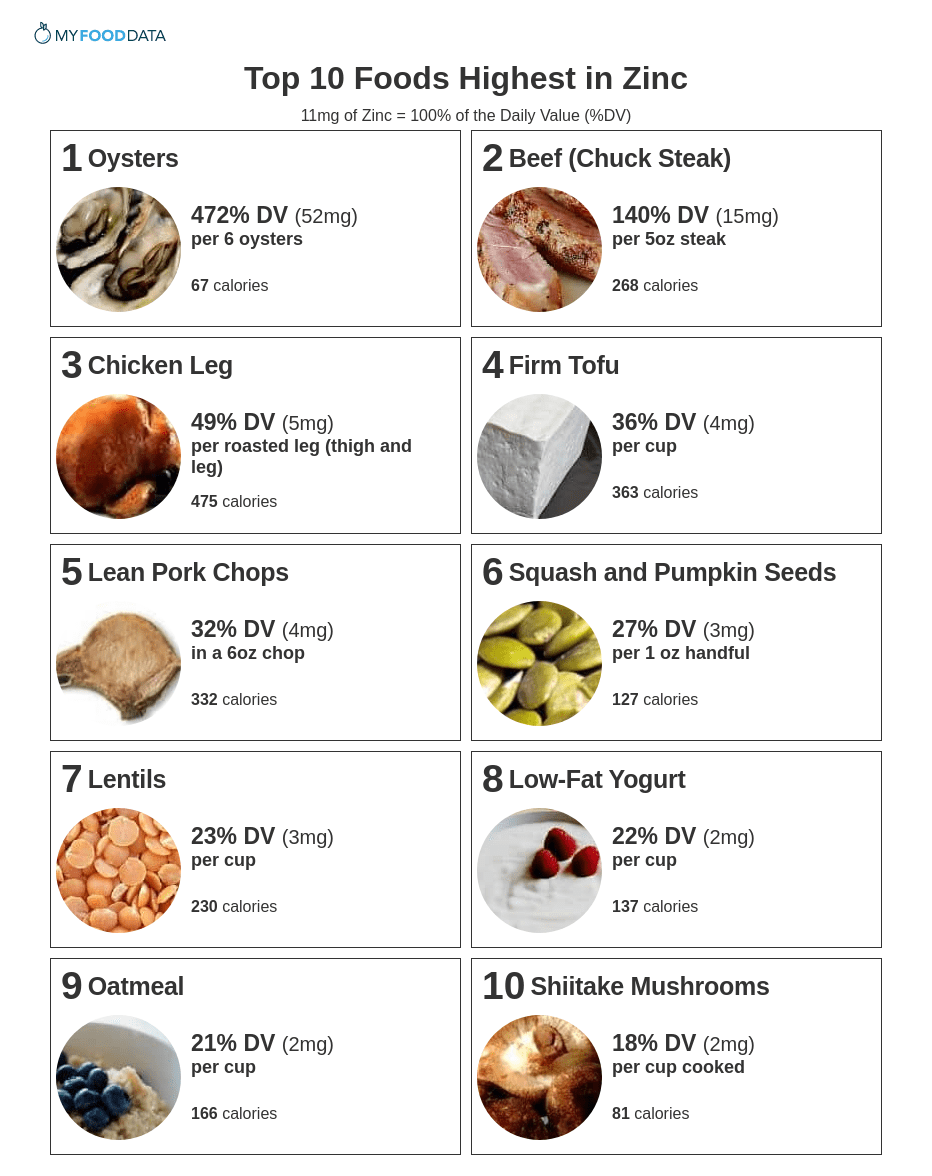The image displays a detailed food data graph titled "Top 10 Foods Highest in Zinc," sourced from MyFoodData. It presents an infographic with images of each food item. At the top, it notes that 11 milligrams of zinc is equivalent to 100% of the daily value (DV). The foods are arranged from left to right and top to bottom, listing their zinc content, daily value percentage, and calorie count.

1. **Oysters**: 472% DV per six oysters, 11 milligrams of zinc, and 67 calories.
2. **Beef Chuck Steak**: 140% DV per five-ounce steak, 15 milligrams of zinc, and 268 calories.
3. **Chicken Leg**: 49% DV per roasted leg with thigh, 5 milligrams of zinc, and 475 calories.
4. **Firm Tofu**: 36% DV with further specifics on serving size omitted.
5. **Lean Pork Chops**: 32% DV with further specifics on serving size omitted.
6. **Squash and Pumpkin Seeds**: 27% DV with further specifics on serving size omitted.
7. **Lentils**: 23% DV with further specifics on serving size omitted.
8. **Low-Fat Yogurt**: 22% DV with further specifics on serving size omitted.
9. **Oatmeal**: 21% DV with further specifics on serving size omitted.
10. **Shiitake Mushrooms**: 18% DV per cooked cup.

Each food item is clearly highlighted both by image and by detailed nutritional data, showing how they contribute to daily zinc intake.